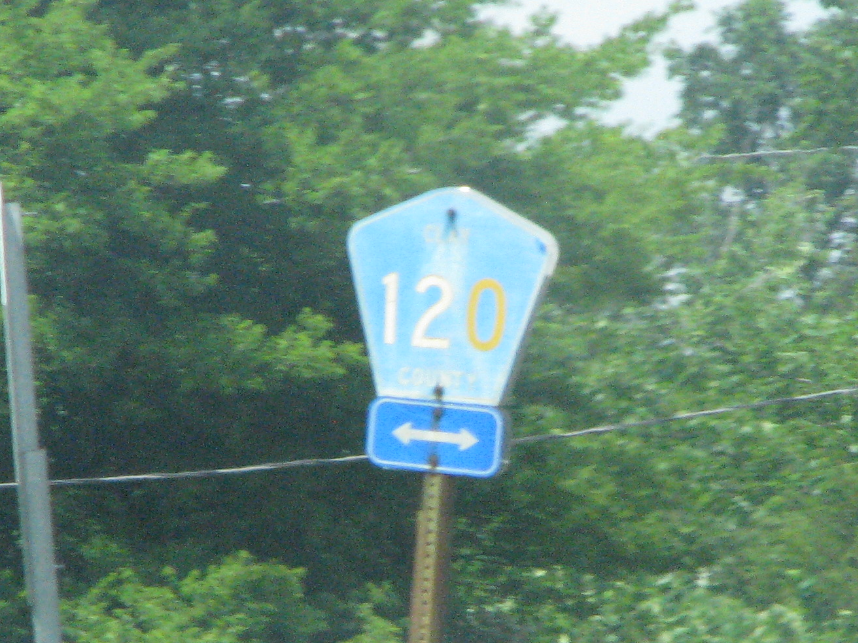The photograph, taken outside, presents a grainy, slightly blurry, vintage feel. Dominating the foreground is a street sign connected to a green to bronze metal pole, secured by rusted screws. The superior sign is shaped like a light blue trapezoid with black rivets at the top and bottom. It displays "Clay County" in white letters, followed by the number 120, with the digits 1 and 2 in white and the 0 in a gold hue. This sign is visibly faded, blending white and blue due to sun exposure. Below it, a second, rounded rectangular sign is attached, featuring a bright blue background with a white border. This sign has two white arrows pointing left and right, indicating a crossroads for Highway 120. The backdrop reveals a dense array of light and dark green trees, partially obscuring the overcast sky with hints of blue. Gray and white lines, possibly telephone or power lines, traverse behind the sign amid the foliage. Another sign, turned away from the camera, is held by a gray pole with additional bracing, adding to the layered complexity of the photograph.